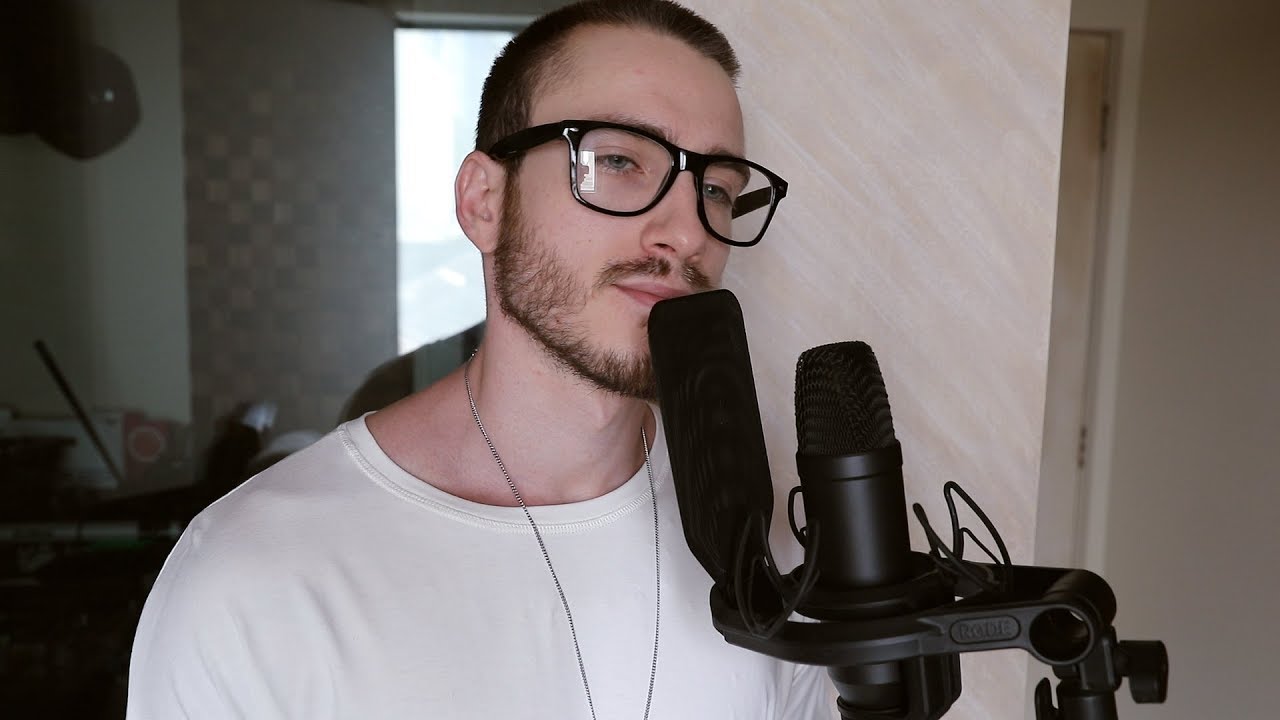A close-up image features a man with short brown hair, wearing black glasses, and sporting a light beard. He is seated at a microphone, with two microphones visible in the shot. One microphone extends from the bottom right side of the image. The man, dressed in a white shirt and accessorized with a long silver necklace, is oriented towards the bottom right corner, showcasing his right side and the front of his face, including his left eye, while his left side remains mostly out of view.

In the background, to the left of the man in the picture (his right side), a door is visible. To the right of the man (the picture's left side), there is a window and the top portion of a lamp in the upper left corner. The scene captures the man in a candid, yet posed moment, emphasizing both his engagement with the microphone and the nuanced details of his surroundings.